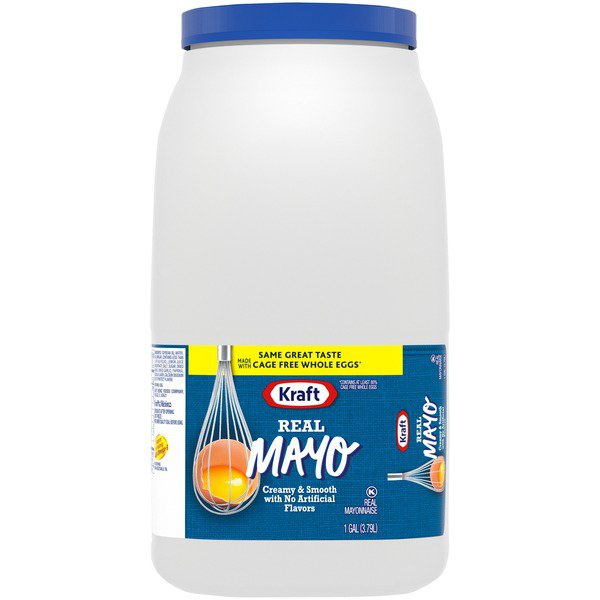The image showcases a tall, white plastic bottle of Kraft Real Mayonnaise with a distinctive blue lid. The label, positioned unusually towards the base, prominently displays the brand name "Kraft" in blue letters within a white background outlined in red. Below it, "Real Mayo" is inscribed, with "Real" in a standard typeface and "Mayo" in cursive. The label also highlights the product's creamy and smooth texture and assures consumers of no artificial flavors. Noteworthy details include a yellow bar above the logo, which reads "Same great taste made with cage-free whole eggs" in black text. Additionally, the design features a whisk holding an egg yolk, accentuating the ingredient quality. The label is more compact than typically seen, covering only the bottom third of the bottle, which is a one-gallon container. On the left-hand side, part of the back label is visible as it wraps around the bottle.